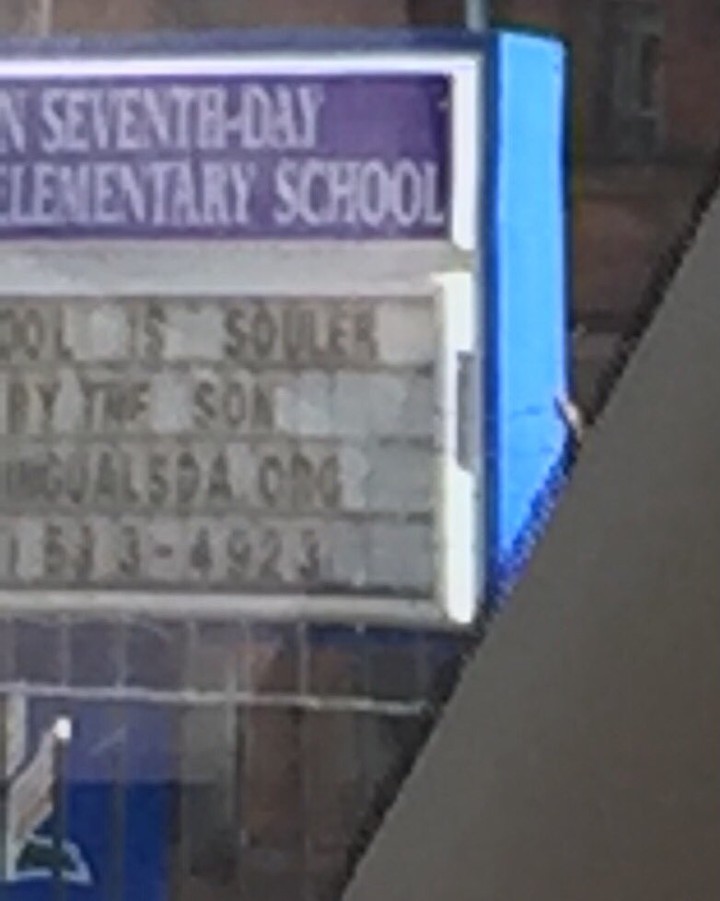This portrait-oriented, slightly out-of-focus photograph features the facade of a church school. Dominating the composition from the center bottom to about three-quarters of the way up on the right side is a black partition, likely a structural element. Inside this partition, there's a prominent three-dimensional sign reminiscent of those typically displayed on church fronts. The sign is framed in blue and consists of two main sections: a smaller blue rectangle at the top with white lettering, and a larger bottom rectangle with black lettering on a white background.

Upon closer inspection, the top section of the sign reads, "Seventh Day," followed by the words "Elementary School" on the next line, indicating it might be the Seventh Day Adventist Elementary School. The bottom section of the sign partially reads, "OOL is Savior by the Sun," followed by additional information including a ".org" website address and a phone number. The sign provides essential details about the institution, despite the image's slightly blurred quality.